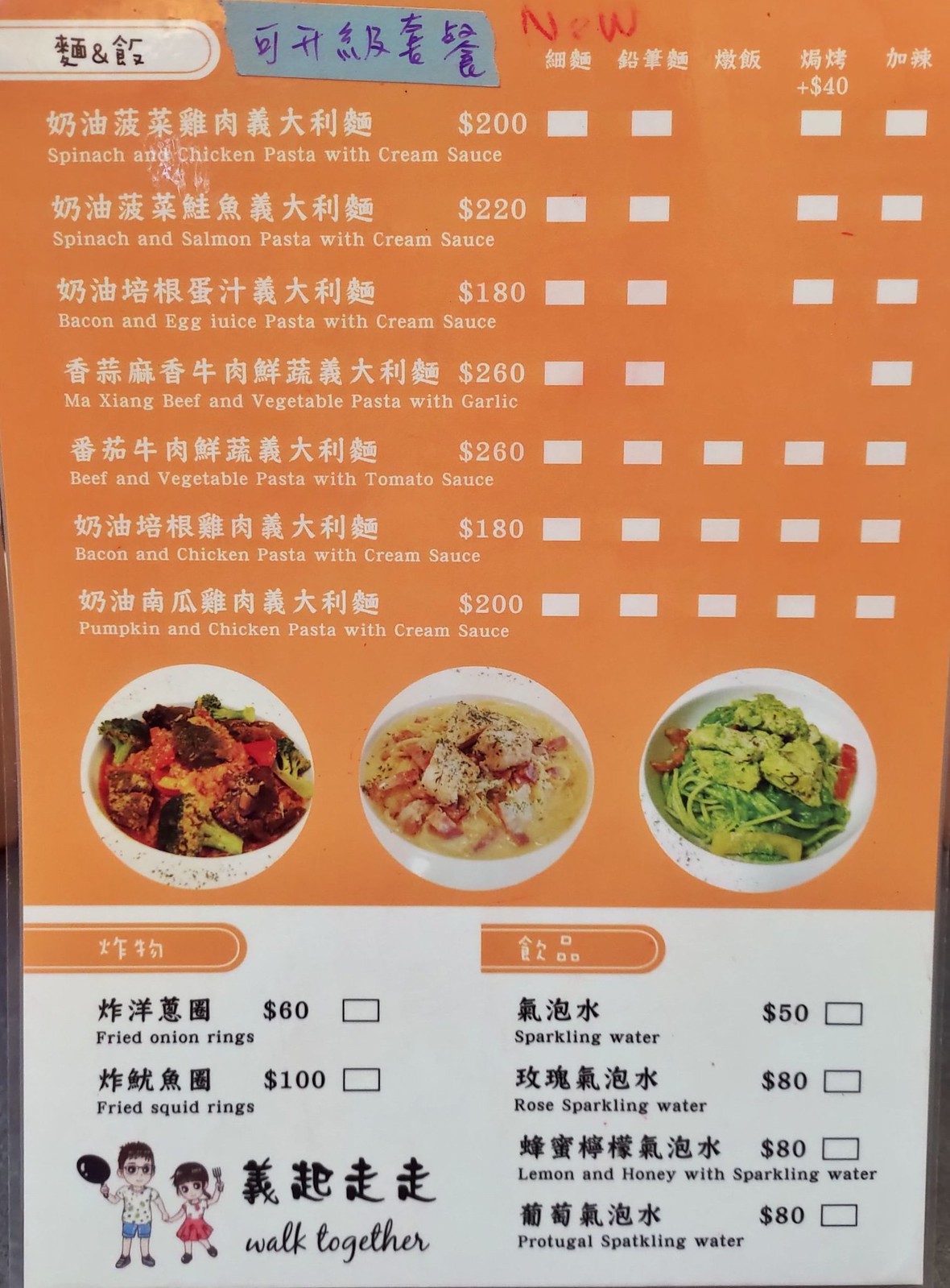**Detailed Caption for Image of Menu:**

The image features a visually striking menu predominantly written in Chinese, with English descriptions provided beneath each Chinese entry. The menu offers a variety of pasta dishes priced at 200 units of an unspecified currency. The first entrée is "Spinach and Chicken Pasta with Cream Sauce," followed by "Spinach and Salmon Pasta with Cream Sauce." Other options include "Bacon and Egg Juice Pasta with Cream Sauce," "Amazing Beef and Vegetable Pasta with Garlic," "Beef and Vegetable Pasta with Tomato Sauce," "Bacon and Chicken Pasta with Cream Sauce," and finally "Pumpkin and Chicken Pasta with Cream Sauce."

The layout incorporates various symbols, possibly indicating dietary considerations such as spiciness or gluten-free options, though some areas are blank. The menu is adorned with photographs of three dishes, showcasing fried onion rings and fried squid rings. The beverage selection includes an assortment of sparkling waters: plain Sparkling Water, Rose Sparkling Water, Lemon and Honey Sparkling Water, and Portuguese Sparkling Water.

The menu’s backdrop is a vivid orange, contrasted by white text. Each food item is presented in white bowls. Adding a whimsical touch, there is an illustration of two children—a boy and a girl—walking together under the words “walk together,” reinforcing a theme of companionship and shared dining experiences.